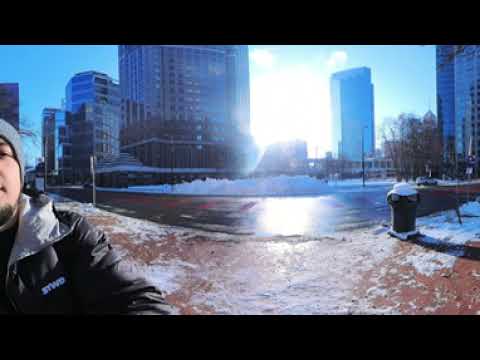In this outdoor scene, the immediate foreground on the left edge of the frame features a young white man with a goatee, wearing a grey beanie and a black jacket with a white lapel. His jacket also has an acronym, "STWD," visible on it. Only half of his body is shown as the image cuts off at his shoulders and chest. Behind him stretches a maroon pavement with patches of snow scattered across it, interspersed with areas where the sunlight gives the appearance of possibly melted snow. A trash can is visible to the right side of the pavement.

Beyond the walkway, there is a road followed by a significant accumulation of plowed snow. The background is dominated by numerous multi-story modern office buildings made of steel and glass, suggesting a cityscape that could be New York City. The sky above is a hazy blue with a bright, indistinct sun illuminating the scene.